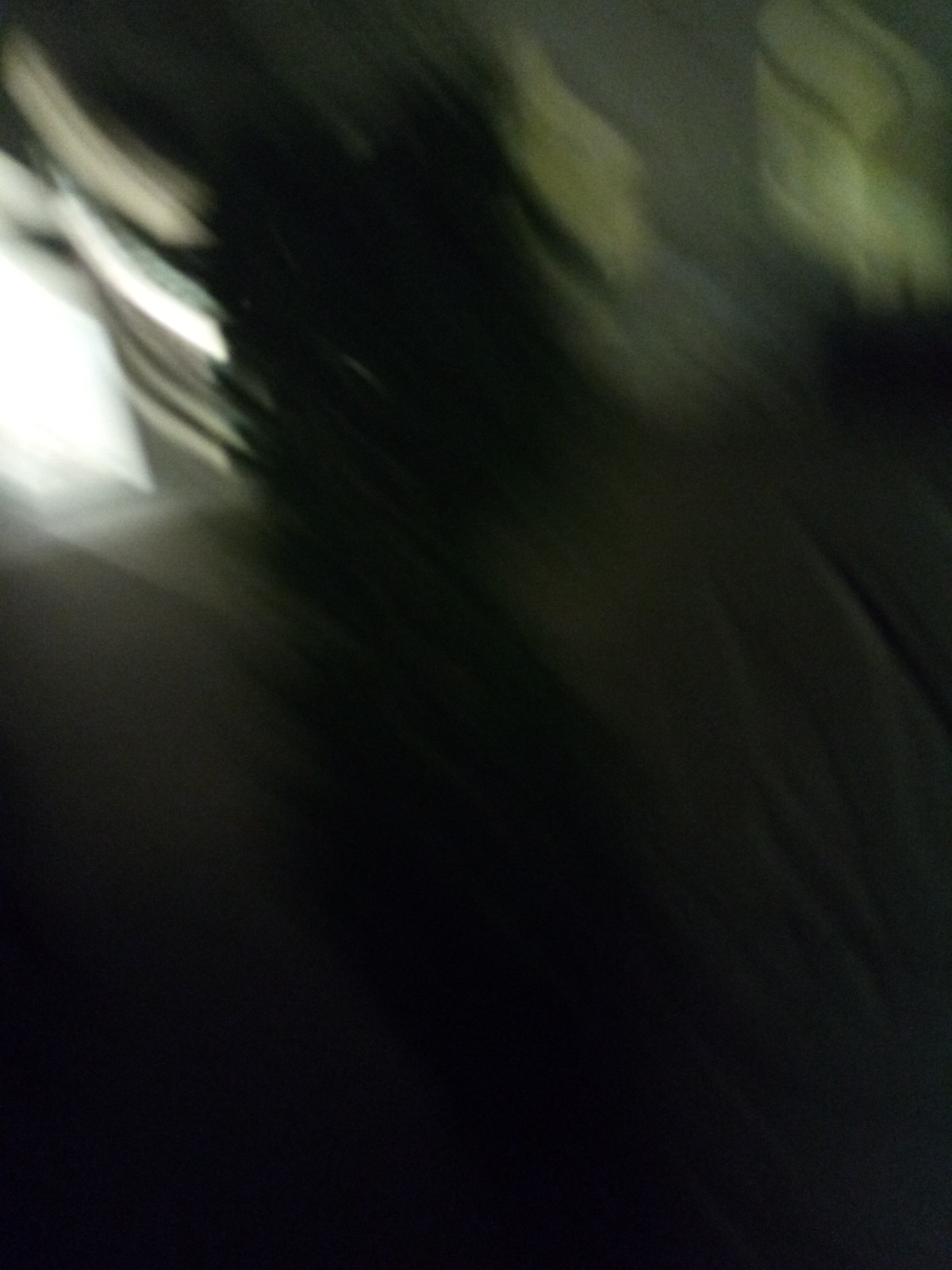This portrait-oriented image is predominantly dark, almost black, with a few areas of light at the top. The brightest portion is a vertical rectangle near the top center, occupying about half the height of the upper section of the image and extending roughly a fifth of the way across from left to right. This bright rectangle resembles a window, with slender horizontal rectangles emanating from its right edge and extending along its top. In the top right corner is another illuminated area, characterized by a grayish-green hue. This section comprises two rectangular shapes: one aligned along the top left edge and the other positioned centrally just left of the image's midpoint.